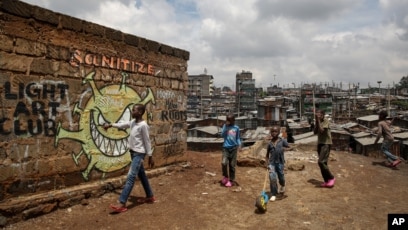This image captures a candid moment in an urban area, likely in Africa, depicting five black children walking and playing on a dirt field. The scene unfolds under a sky heavily obscured by white clouds. In the background, a variety of buildings are visible, resembling a shantytown with small, crudely constructed homes made of random tin and metal materials.

Dominating the left side of the image is a flat red brick wall, adorned with expressive street art. At the top of the wall, in orange letters, the word "Sanitize" is visible, while to the left, "Light Art Club" is inscribed in black letters. Prominently, the wall features a vivid drawing of a green virus cell, likely representing the coronavirus, characterized by its sinister smile and sharp teeth.

Of the five children, all are wearing denim trousers—four in dark blue and one in black. Four of them sport brightly colored red shoes, and one has white shoes. Their upper garments vary, with two dressed in T-shirts and three in long-sleeve T-shirts. One child is engaged with a yellow toy featuring a blue base and a green wheel. The child leading the group is clad in a white shirt and blue denim, walking adjacent to the graffiti-laden wall. In the bottom right-hand corner, the image bears a watermark, "AP," suggesting it is a photograph from the Associated Press. 

This evocative scene, steeped in the daily life of its young subjects and rich in environmental details, paints a vivid picture of resilience and creativity in a seemingly impoverished urban landscape.